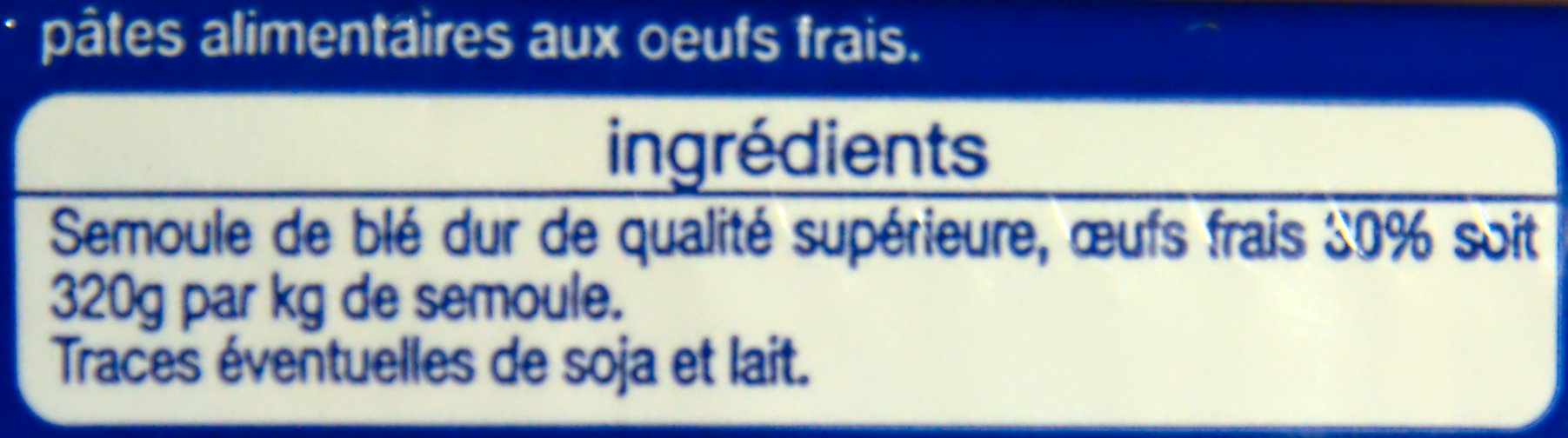The image depicts a blue-colored food label showcasing detailed information in French. The label is segmented into two main areas: the upper part has a blue background with white text that reads "Pâté alimentaire au frais," which may refer to fresh food or fresh pâté. Below this, there is a white section with blue text that lists the ingredients in French. The ingredients include terms like "amour de bleu," which suggests a love of blue or blue cheese, "de qualité supérieure," implying superior quality, and "au frais," indicating that the product is fresh. It also mentions "30%," likely denoting the percentage of a specific ingredient, and "320 grams," implying the weight of the product. The label emphasizes the premium quality and freshness of the ingredients used.